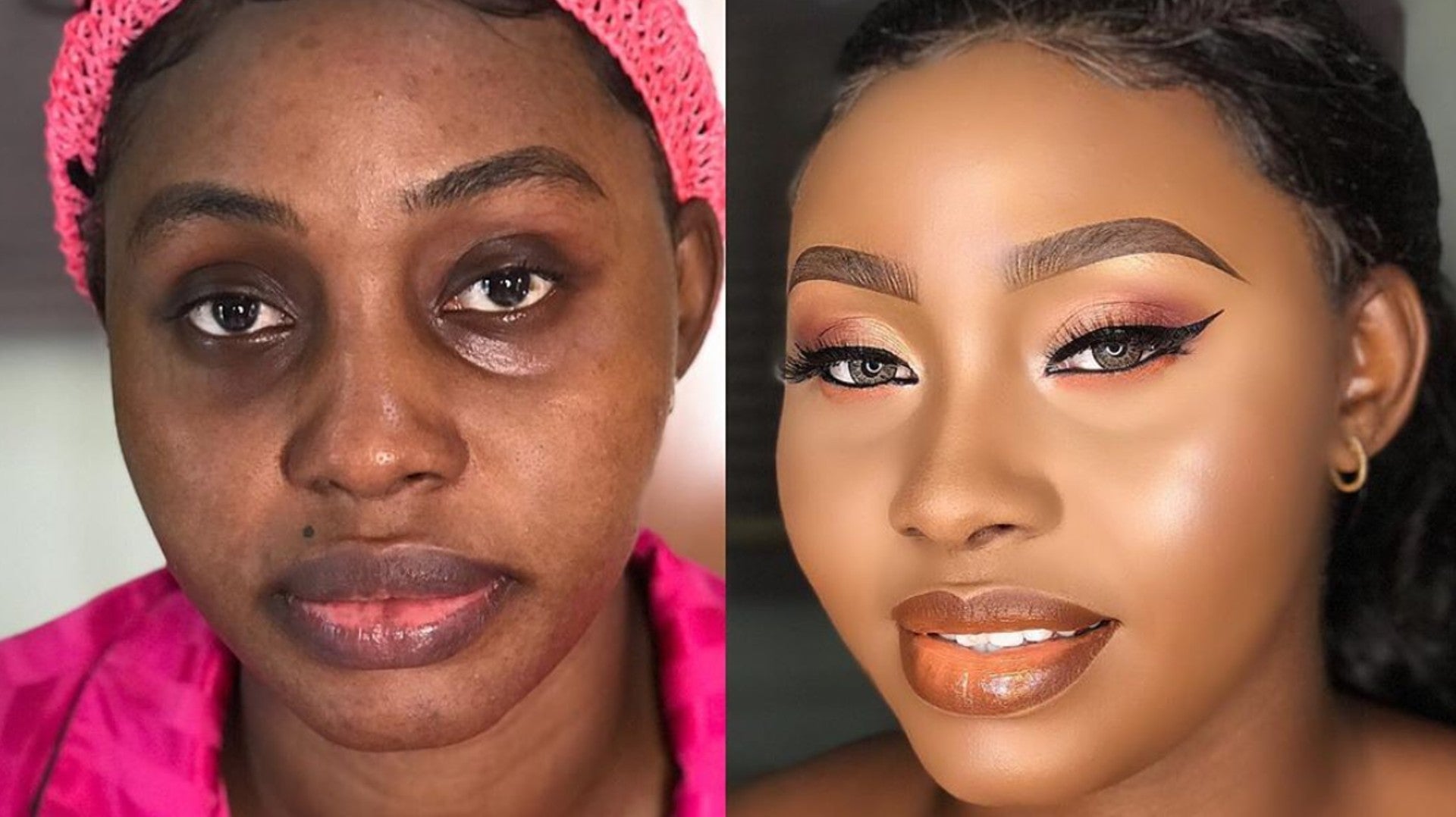This image features a striking transformation portrayed through two side-by-side photos, possibly suggesting a makeup tutorial or a "before and after" comparison. Both images depict a dark-skinned woman with subtle variations in her appearance.

In the left image, the woman wears a pink bonnet and a pink pajama top or nightgown. Her natural complexion showcases her beautiful dark skin adorned with some blemishes and a mole above her lip. Her lips exhibit a unique two-tone look, with a darker shade on the outer part and pink on the inner portion. Her eyes have some dark circles, indicative of a tired expression, and her skin appears slightly oily. She does not appear to be wearing any makeup.

The right image dramatically shifts the focus with the same woman now lightened in skin tone, presenting a smooth and glowing complexion free of any blemishes. This polished look is augmented with orange eye shadow, black eyeliner, and meticulously penciled eyebrows. She sports false lashes, giving her eyes a captivating cat-eye effect. Her lips now bear a glossy, darker brown hue with the pink interior still visible. Adding to her refined look, she wears a small hoop earring. Her poised expression, with lips slightly parted to show her white teeth, enhances her overall polished and glamorous appearance.